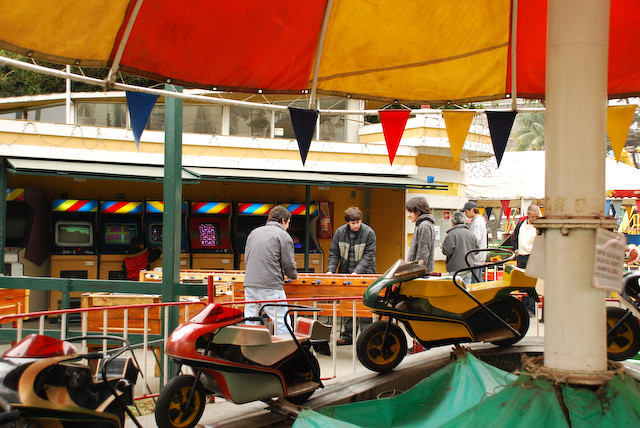This photograph captures a vibrant scene at a carnival, with a focal point on a carousel-style amusement ride featuring stationary toy motorcycles instead of traditional horses. In the very forefront, three visible motorcycles in distinct colors—yellow and green in the center, white and red to the left, and partially cropped white and gray to the bottom left—add a playful splash of color. The central axis of the ride is marked by a tall, cylindrical white pole situated towards the right of the image, supporting a large, umbrella-like canopy above. This canopy, segmented in alternating yellow and red sections, stretches horizontally across the top of the image. Beneath it dangle triangular pennants in an alternating mix of blue, yellow, red, and black.

In the background, there is a lively setup featuring various carnival activities. A group of teenage boys are engaged in a game of foosball at a light brown wooden table, appearing engrossed in their play. Behind them, six to eight arcade machines line up under a white canopy, adding a nostalgic touch with their glowing screens partially obscured by the foosball players. Further back, the scene shows at least three other carnival-goers strolling around and partaking in the festivities, with another umbrella visible to the right and a palm tree partially obscured by the central white pole. The background also includes semi-obscured men who may be workers, hinting at the bustling nature of the carnival. The ambiance of the image captures the essence of a merry, colorful, and engaging carnival day.